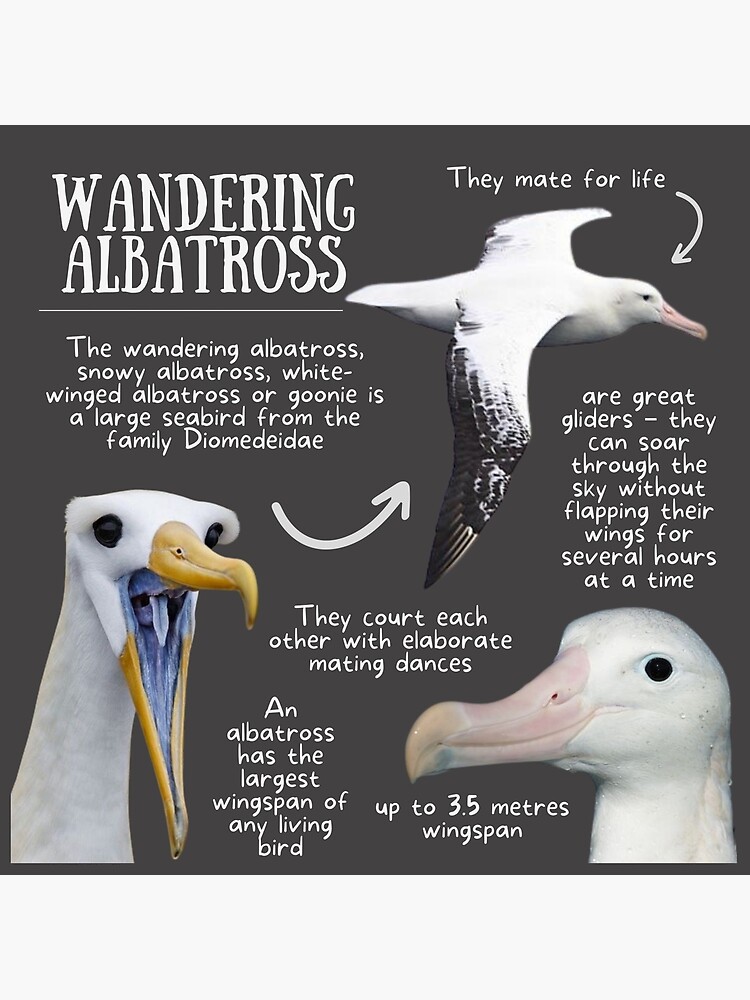This detailed graphic about the wandering albatross (also known as the snowy albatross, white-winged albatross, or goonie) features a photorealistic portrayal with three distinct images of the bird in various stages. Set against a charcoal background, the graphic's heading in white letters reads "Wandering Albatross." Below it, descriptive text outlines that the wandering albatross is a large seabird from the family Diomedidae. 

One key image shows the albatross in mid-flight, highlighting its impressive white plumage with black-tipped wings, alongside a note mentioning their ability to glide for hours without flapping their wings. Another image captures a close-up, frontal view of the bird with its beak gaping open, either as part of an elaborate mating dance or a signal of hunger. This image reveals a long yellow beak, beady black eyes, and a blue-tinted interior of the mouth. A third accompanying image features the bird's head, emphasizing its record wingspan of up to 3.5 meters.

Throughout the graphic, informative tags point out that these birds mate for life and court with elaborate dances, encapsulating the awe-inspiring biology and behavior of the wandering albatross.